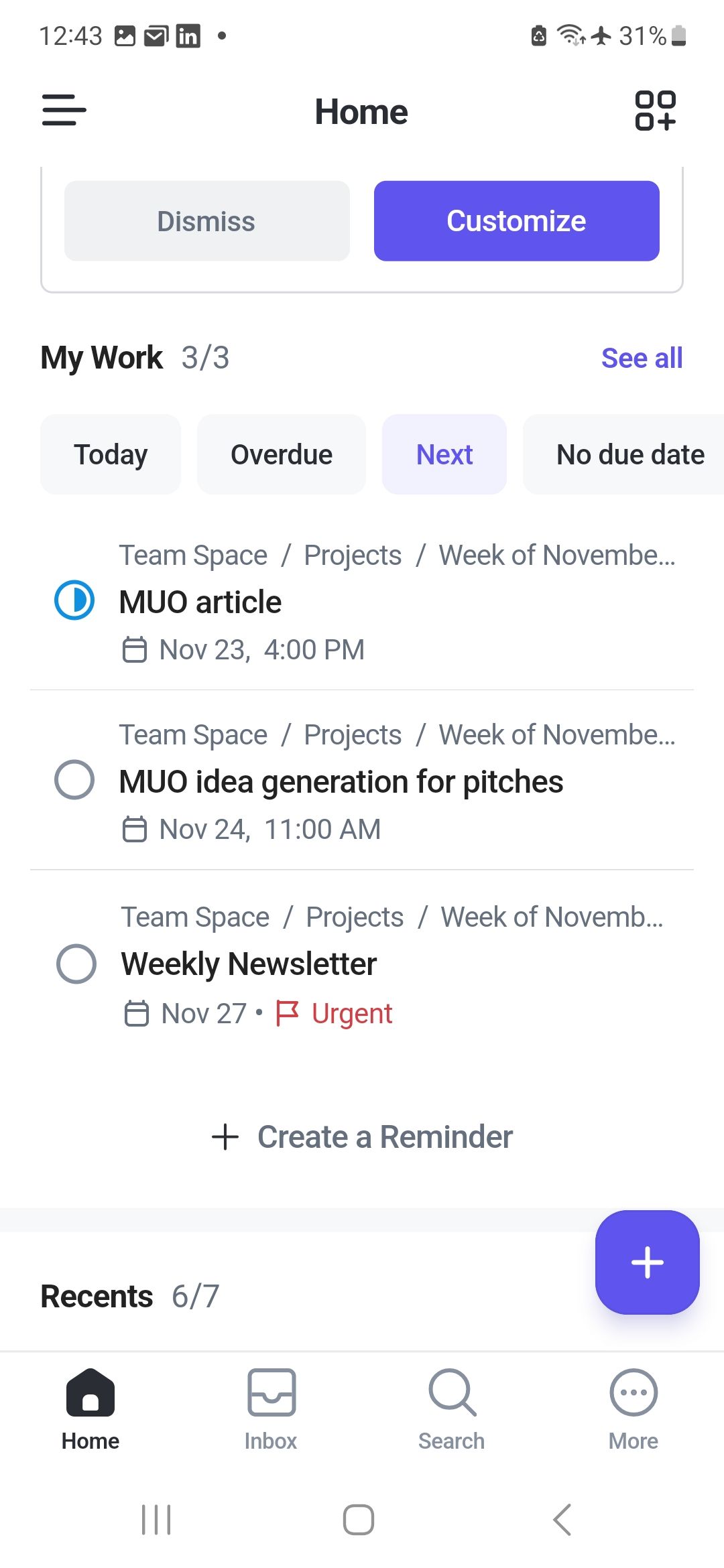A screenshot from a smartphone displaying the time "12:43" at the top left and the battery level at "31%" in the top right corner. Below this, the word "Home" is centrally positioned. There are two buttons below that: a gray "Dismiss" button on the left and a purple "Customize" button on the right. Further, the screen shows "My work: 3 out of 3" with a "See All" option on the right side. Below, there are four buttons labeled "Today," "Overdue," "Next," and "No Due Date." At the bottom of the screen, gray text reads "Team Space / Project / Week November," followed by a round blue icon featuring a half-moon symbol. Next to the icon, "MUO Article" is written in black text, with a calendar icon and "November 23rd at 4 p.m." in gray text below.